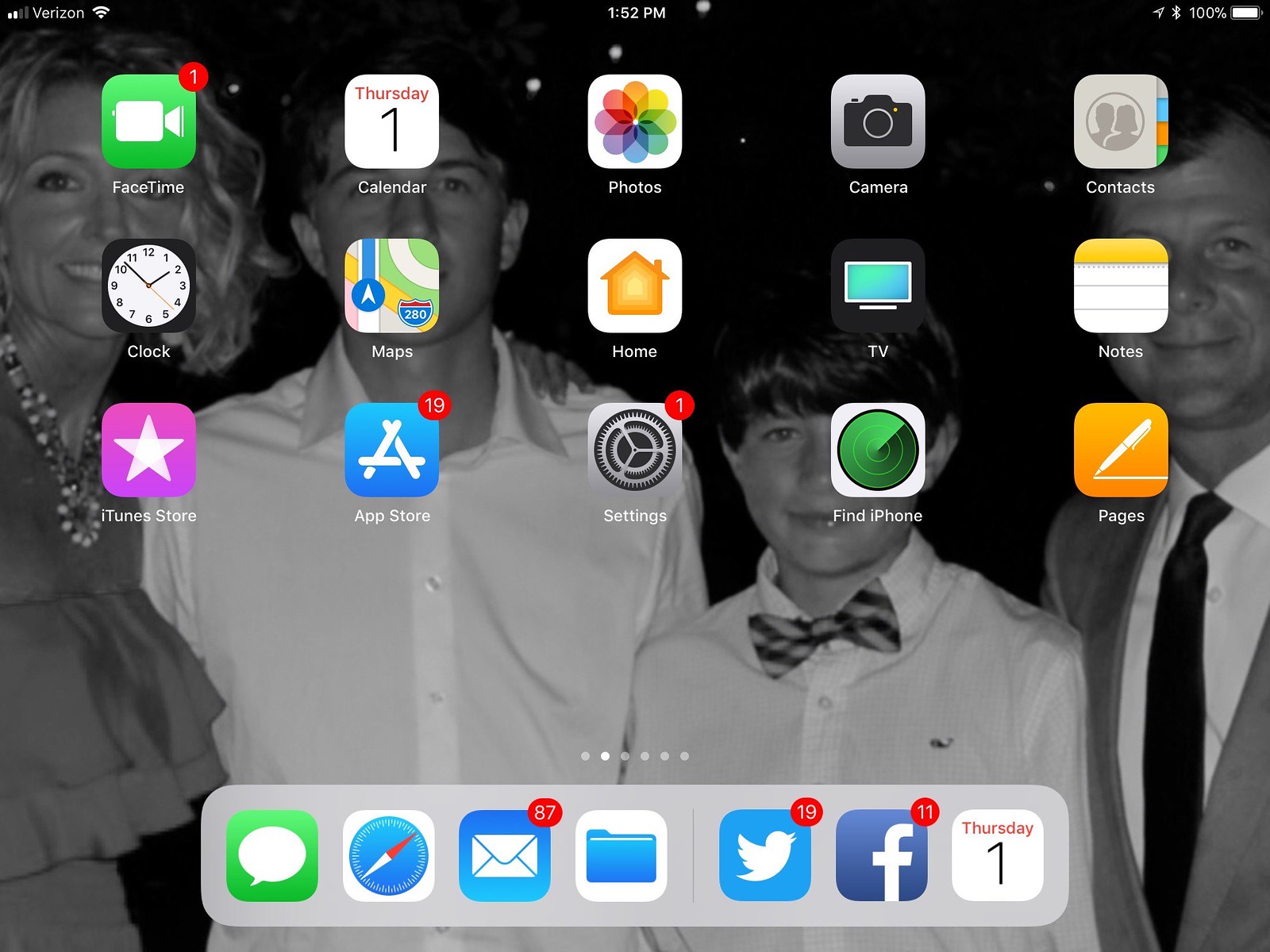The image showcases a tablet's home screen in a wide rectangular format. The background wallpaper is a black-and-white photograph of a family. On the left side of the photo is a blonde woman adorned with a beaded necklace, smiling warmly. In the center are two young men, both dressed in white shirts; one of them sports a bow tie. To the right stands a man clad in a gray suit jacket, paired with a white shirt and a long, slim black tie. 

The home screen displays several colored app icons organized in three rows, including FaceTime, Calendar, Photos, Camera, and Contacts. At the top of the screen, the Verizon network signal is visible, the time reads 1:52 p.m., and the battery indicator shows a full charge at 100%.